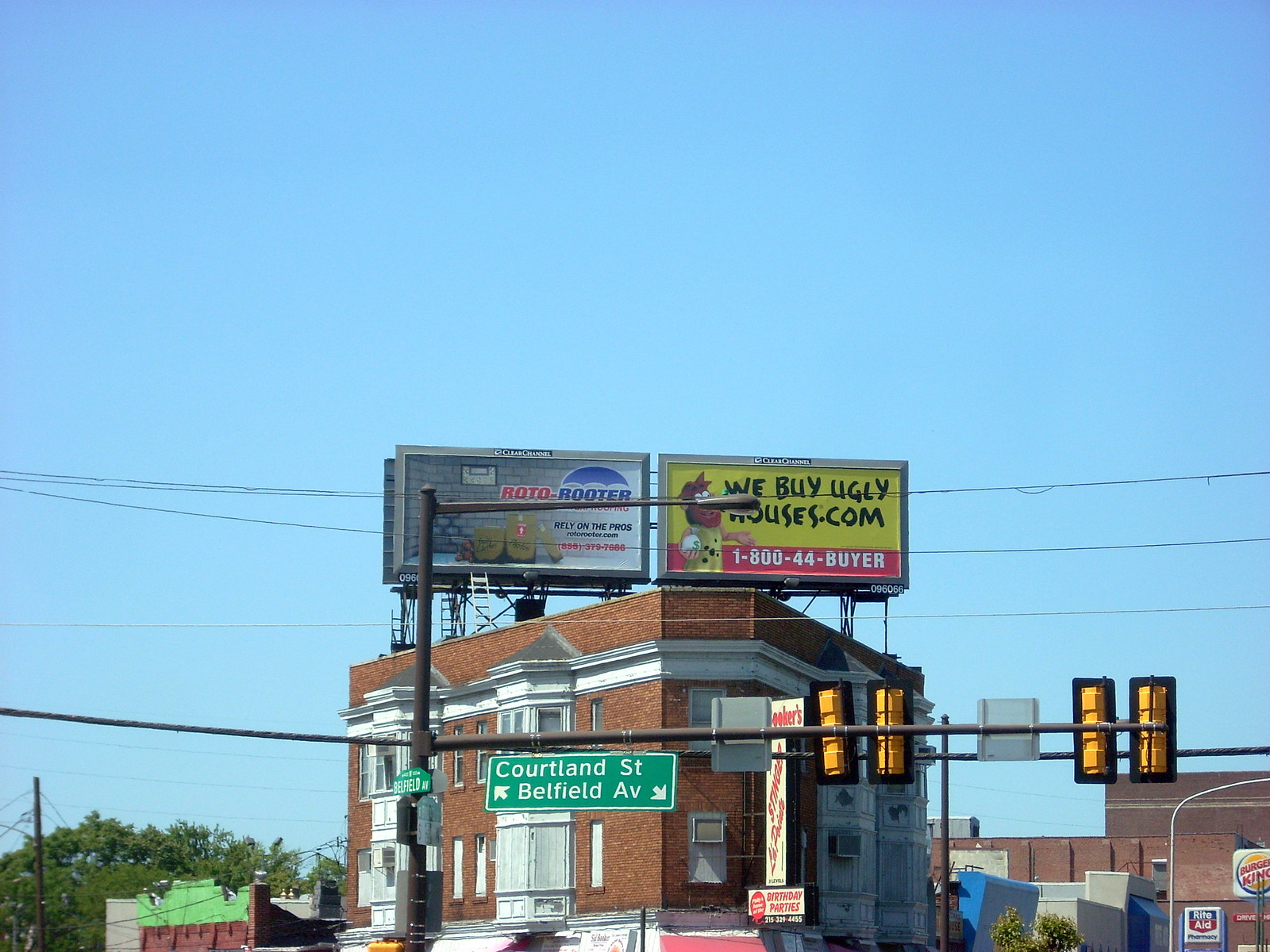A clear blue sky forms the backdrop of the image, intersected by a crisscross of electrical wires extending horizontally across the frame. In the bottom left corner, green leaves add a splash of natural color to the scene. Further down, much lower in the frame, is a green street sign with white text indicating "Portland Street" and "Bellevue Avenue." Above this sign, and to the left, the backside of a traffic light, predominantly yellow with black casing, is visible. 

On the left side of the image, a black-and-gray sign reads "Roto-Rooter." To the right of this sign is a yellow banner with black text promoting "WeBuyUglyHouses.com," accompanied by a graphic of a person in red. Below this banner is a white rectangle with red text displaying the phone number "1-800-44-BUYER." 

These signs appear to be mounted on the side of a brick building featuring several white-framed windows. Additionally, there is a sign extending perpendicularly from the building’s facade, showing more red text on rectangular backgrounds. At the very bottom right of the image, logos for Burger King and Rite Aid are faintly visible, adding to the urban commercial context of the scene.